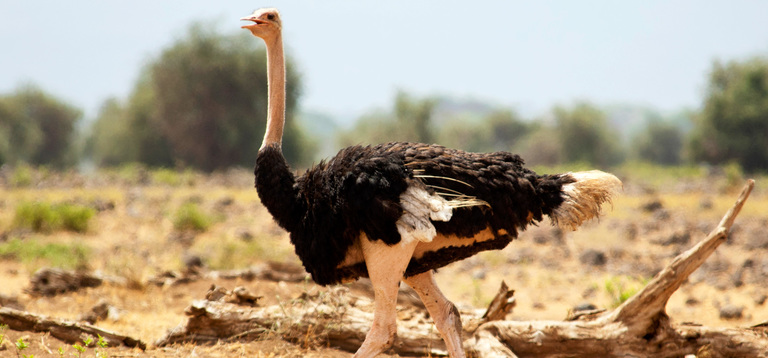In this detailed image, a tall, striking ostrich with a long, thin grayish-white neck and a mixture of black and white feathers is captured mid-movement with its mouth open, seemingly trying to cool off on a hot day. The ostrich has black eyes, a yellowish beak, and trots on long, sturdy legs. It appears to be walking in a dry riverbed or lakebed filled with various natural elements. The ground is a yellowy-brown dirt with scattered black rocks and a few small, green bushes. Prominently, there are bleached, downed trees and logs which the ostrich is navigating over. In the backdrop, a stark contrast is created by large, bushy trees, a mixture of green and brown hues, while the sky is an unusual gray, leaning towards white, indicating the harsh sunlight. The overall scene radiates the impression of arid, sun-soaked terrain.